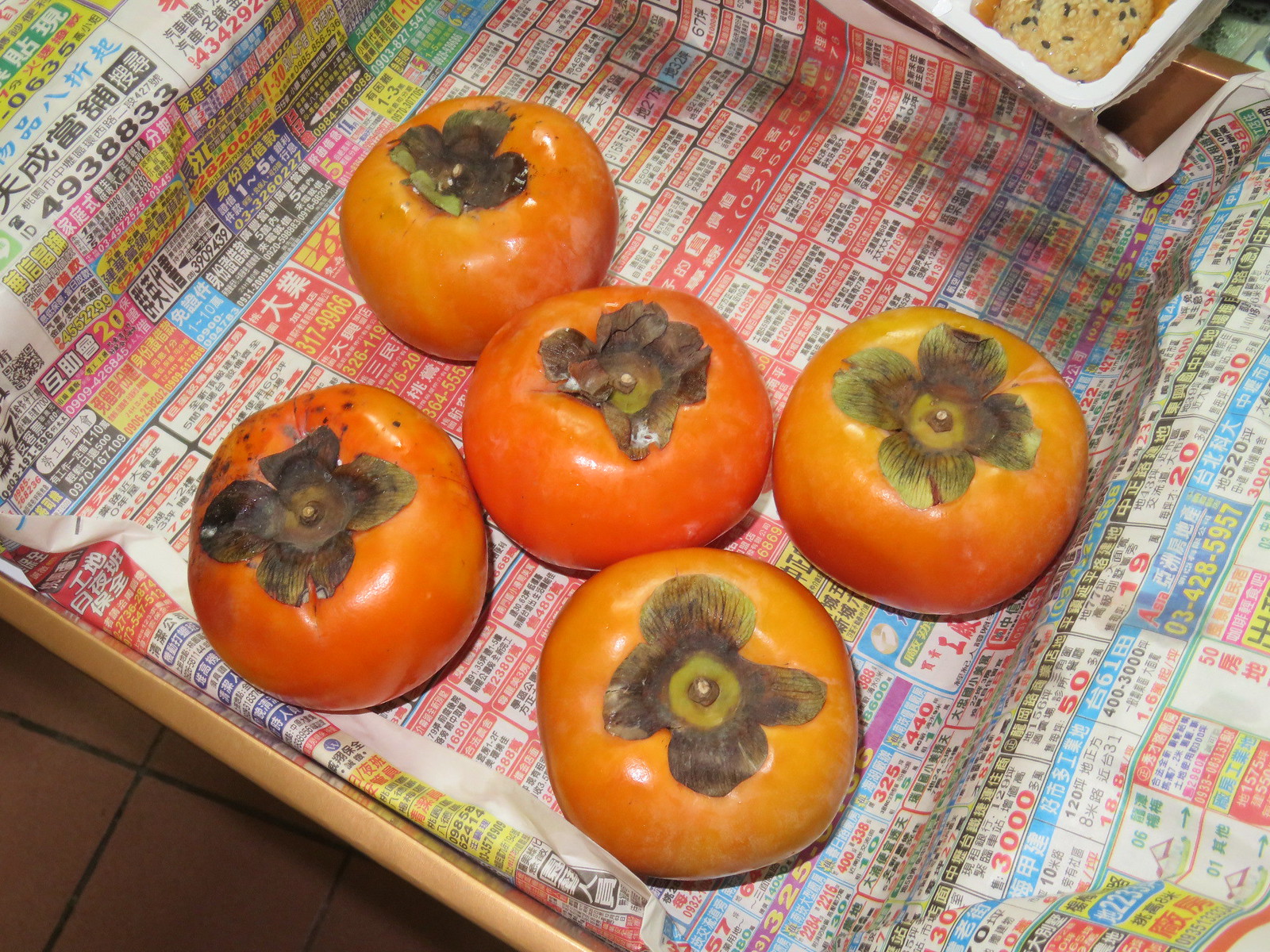The image is a color photograph featuring five ripe persimmons, arranged in a formation where two are on the left, two on the right, and one in the center. These persimmons are of the large Japanese variety, displaying a gradient of red hues, with the central persimmon appearing slightly darker than the others. They rest on a piece of newspaper with Japanese or Chinese characters, with vibrant blocks of red, blue, white, and black interspersed. This newspaper lines a light brown tray, which sits on a tan countertop or floor with dark grout lines. In the top right corner of the image, there is a white plastic food container, possibly holding rice or shrimp, adorned with black sesame seeds.